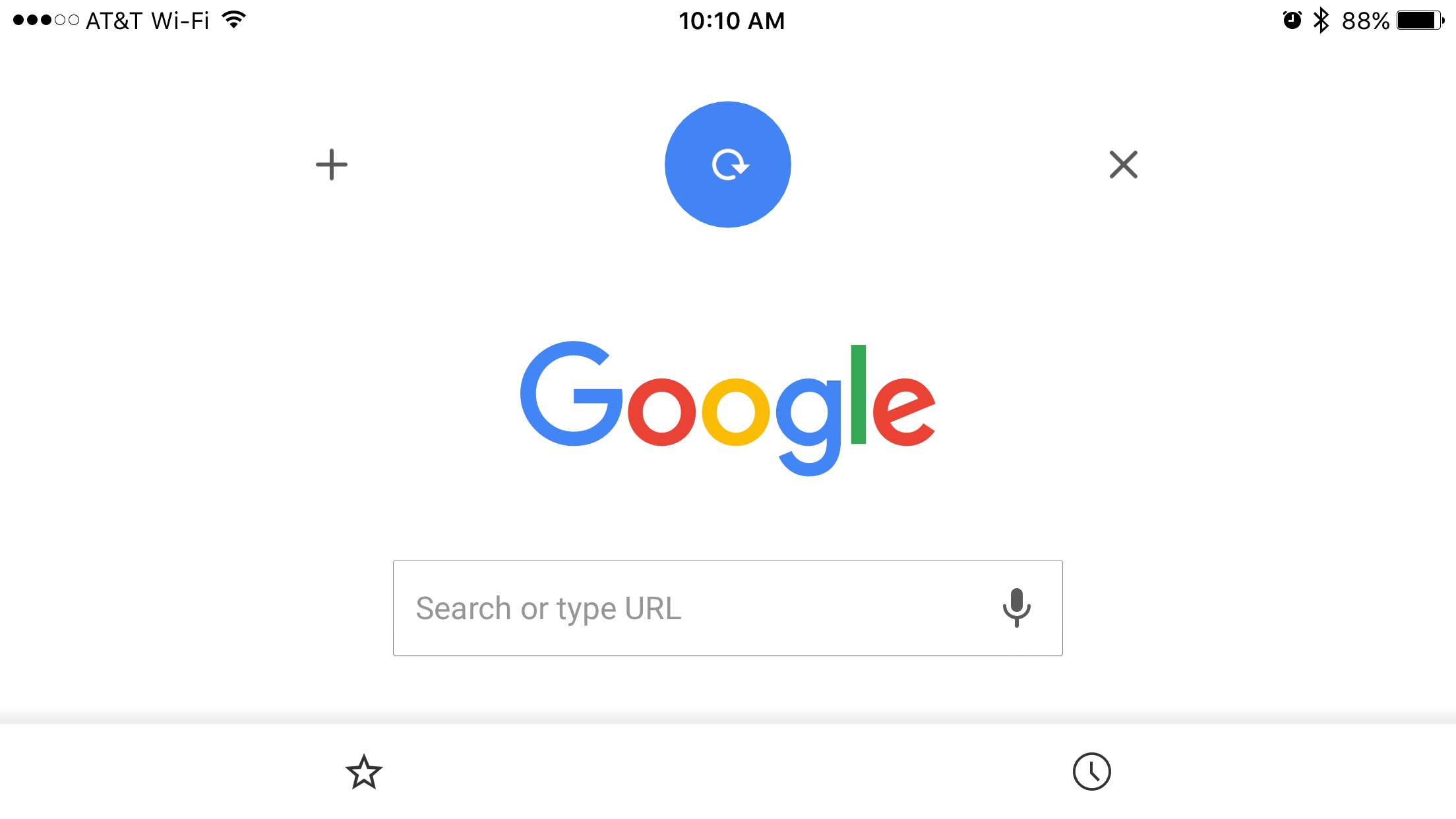This screenshot appears to be taken from an iPad, as indicated by the dimensions and various UI elements visible. The top left corner displays "AT&T Wi-Fi" along with the Wi-Fi icon, showing three out of five filled dots. Centrally, the time is displayed, reading 10:10 AM. On the right side, there are icons for an alarm clock, Bluetooth, and a battery indicator showing 88% charge.

The screenshot captures the Google homepage with a distinct feature at the top. On the left is a plus sign, on the right is an X, and between them, Google's logo is prominently displayed. Above the Google logo, there's a circular blue button with a replay arrow, suggesting it might be part of a special Google Doodle. Below the logo, a search bar reads "search or type URL." Additional smaller icons, a star, and a clock are also visible, indicating bookmark and history functionalities, respectively.